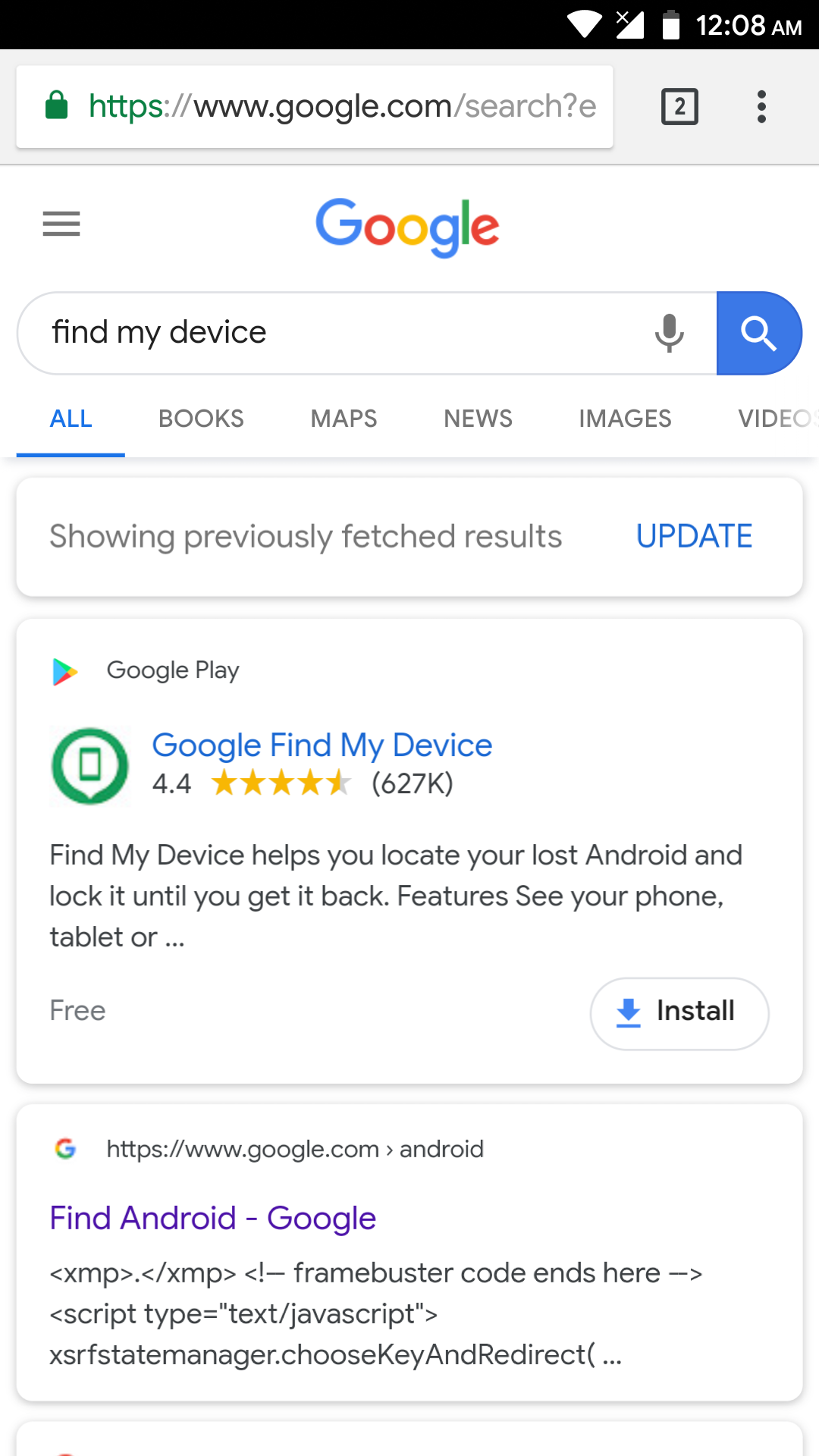**Screenshot Details of Google Search for "Find My Device" on an Android Device**

This screenshot captures the Google app interface on an Android device, displaying the user's search results for "Find My Device." The search was conducted at 12:08 AM, with the device connected to WiFi but showing no cellular service bars. The battery indicator reveals that the device's battery is just below full, likely above 50%.

The search results include:

1. **Google Find My Device App**: 
   - The first result prominently features the "Google Find My Device" app available on Google Play.
   - The app boasts a rating of 4.4 stars from 627,000 reviews, denoting its popularity and reliability.

2. **Find Android**:
   - The second result is a link to the "Find Android" feature, hosted on Google's website.
   - The link appears in purple font, indicating it has been previously visited by the user.

This detailed screenshot provides insight into both the search process and the status of the user's device at the time of capture.